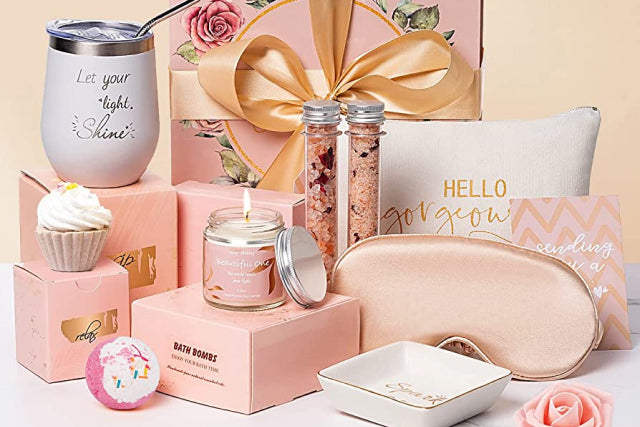This image showcases an elaborate spa-themed gift set, arranged against a pink backdrop with a large pink card in the center adorned with a gold bow. The card features a pink circle with gold trim and floral details. To the left, a white insulated mug with the phrase "Let Your Light Shine" in silver, and a metal straw sticking out, sits atop a pink box. Directly in front of this is a smaller pink box displaying a white cupcake.

A pink ball, resembling a bath bomb with frosting and sprinkles, sits in front of the cupcake box. To the right, another pink box supports a lit glass candle, its lid leaning against the base. Behind the candle's box, the top edge of yet another box can be seen. Centered to the right, two glass tubes filled with pink crystals and topped with silver caps put forth a delicate aesthetic.

Adjacent to these, a white pillow, bearing "Hello Gorgeous" in gold lettering, shares space with a pink eye mask lying halfway down its front. Behind and slightly overlapping the eye mask is a card with pink and gold zigzags, though its text remains unreadable. Below the mask, a white dish with gold trim holds a pink rose in its corner.

This thoughtfully designed gift set, which includes elements like bath bombs, candles, and spa accessories, embodies a luxurious and relaxing experience perfect for self-care.